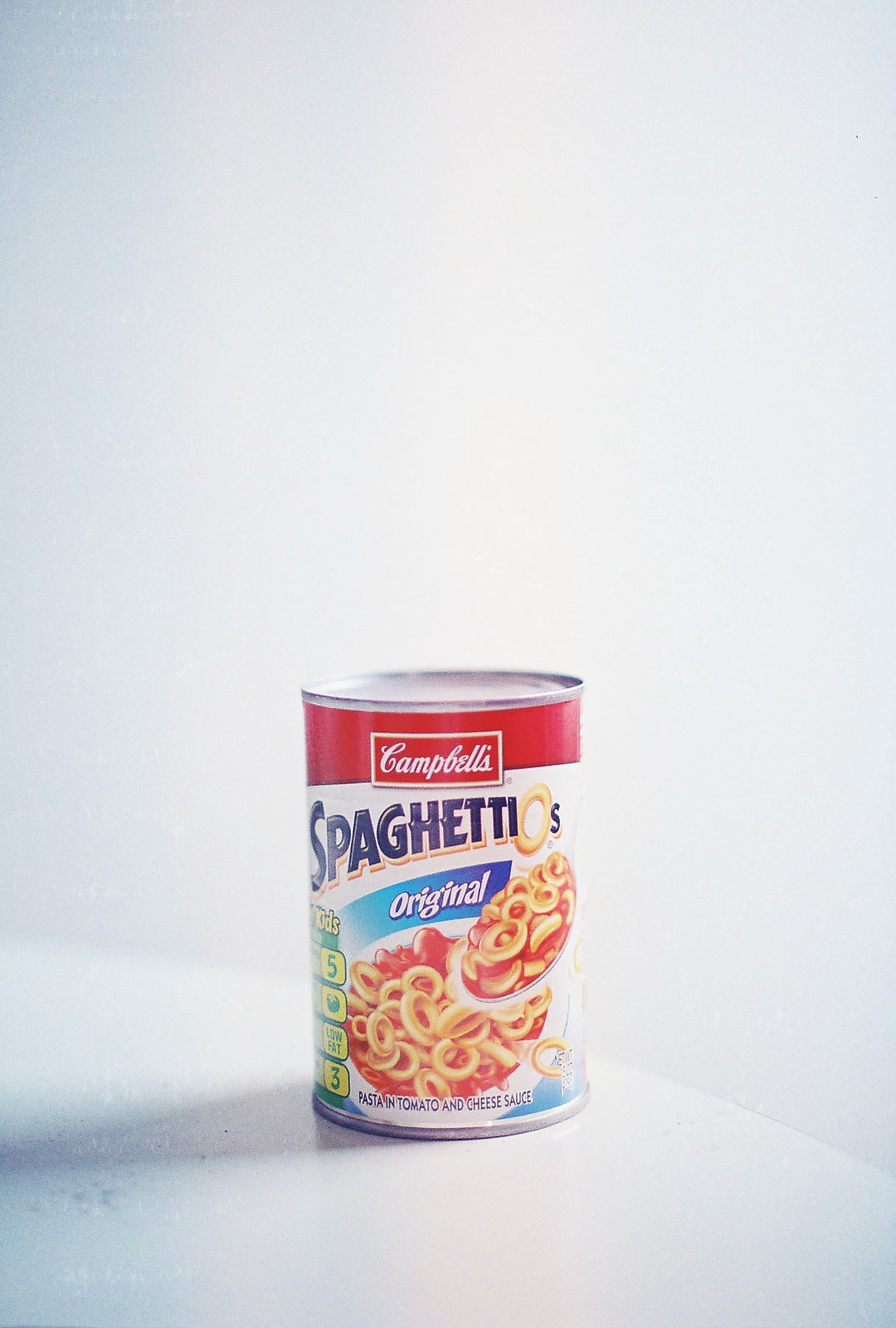This is a detailed and vibrant stock photograph of a can of Campbell's SpaghettiOs Original. The can is set on a white circular table with a matching white background, illuminated by artificial light, casting a shadow to the left. The can itself is a standard soup can size with a silver top, lacking a pull tab.

The label design is striking and patriotic, featuring bold colors and detailed elements. At the top, the iconic Campbell's logo is presented in white cursive within a red rectangle background. Below this, the word "SpaghettiOs" is boldly printed in black, with the characteristic 'O' doubling as a piece of pasta. Beneath that, the term "Original" is showcased in white letters against a royal blue banner. 

An appetizing image on the lower part of the can displays a bowl of SpaghettiOs in tomato and cheese sauce, with a ladle filled with the circular pasta dipping into the bowl. Nutritional information is partially visible on the left side of the label, marked by yellow highlights. The label is primarily white, complementing the overall clean and simple aesthetic of the photograph.